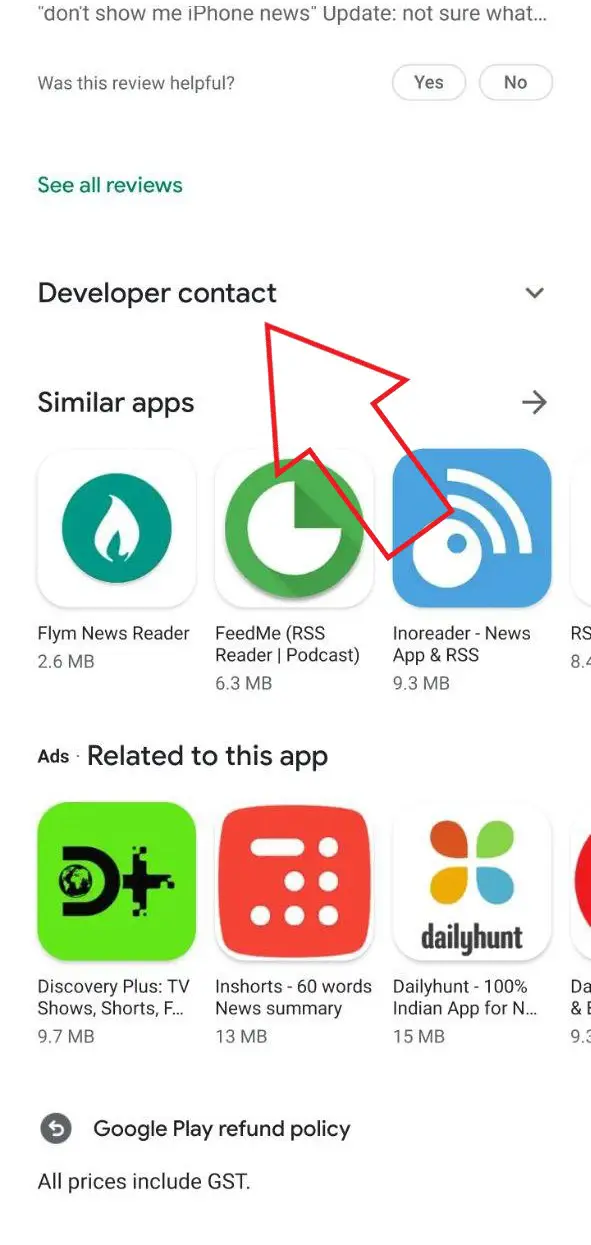The image features a white background with various elements typically found in an app review interface. At the top, there is a message reading "Don't show the iPhone news update," though the context is unclear. Below this, the phrase "Was this review helpful?" is prominently displayed, accompanied by "Yes" and "No" buttons.

Further down, "See all reviews" is written in green text. Next to it, there is a "Developer contact" option with a down arrow. A large red arrow points upward towards the "Developer contact" section, emphasizing its importance. Additionally, there is a "Similar apps" section with a right-facing arrow, guiding the viewer to related applications.

Highlighted apps in this section include:
- Flynn Newsreader
- Feed Me, RSS Reader Podcast
- Increter News app and RSS

The image also includes a segment labeled "Ads related to this app," showcasing:
- Discovery Plus, TV shows
- In short, 60 words news summary
- Daily Hunt, 100% Indian app

In the bottom corner, there is a partially visible red circle and a smaller gray circle with a turnaround arrow, indicating the Google Play refund policy. The text at the bottom notes, "All prices include GST."